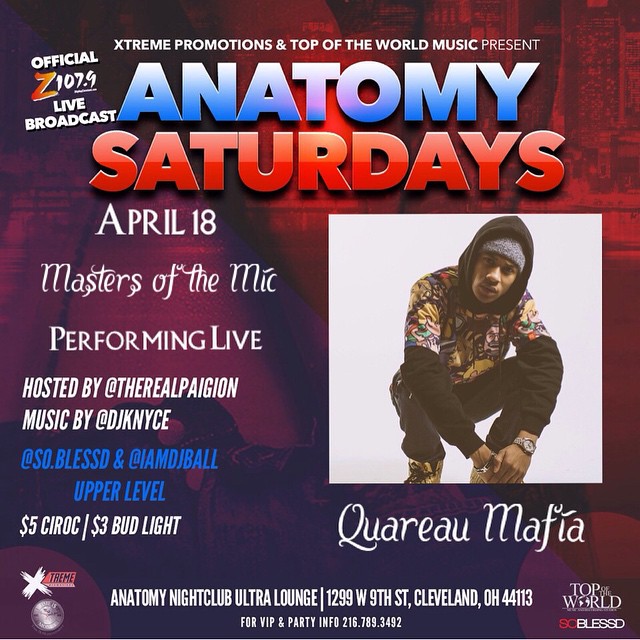This image is a digitally made advertisement with a red, blue, white, orange, and yellow color scheme for an event called "Anatomy Saturdays," taking place on April 18th at Anatomy Nightclub Ultra Lounge, located at 1299 West 9th Street, Cleveland, Ohio, 44113. It is presented by Extreme Promotions and Top of the World Music, and will be an official Z107.9 live broadcast. The main performance will feature "Masters of the Mic" performing live, and the event will be hosted by The Real Pie Gone. Music will be provided by DJ Nice, So Blessed, and IAMDJBall. On the right side, there's a picture of a man crouched down wearing a colorful graphic hoodie over a yellow shirt and a hat, with a serious expression. His stage name, Quaray Mafia, is displayed beneath his image. Entry prices are listed as $5 for CÎROC and $3 for Bud Light. The flyer also provides VIP and party information, directing inquiries to 216-789-1349. Multiple logos for the promoters and sponsors are scattered across the image.